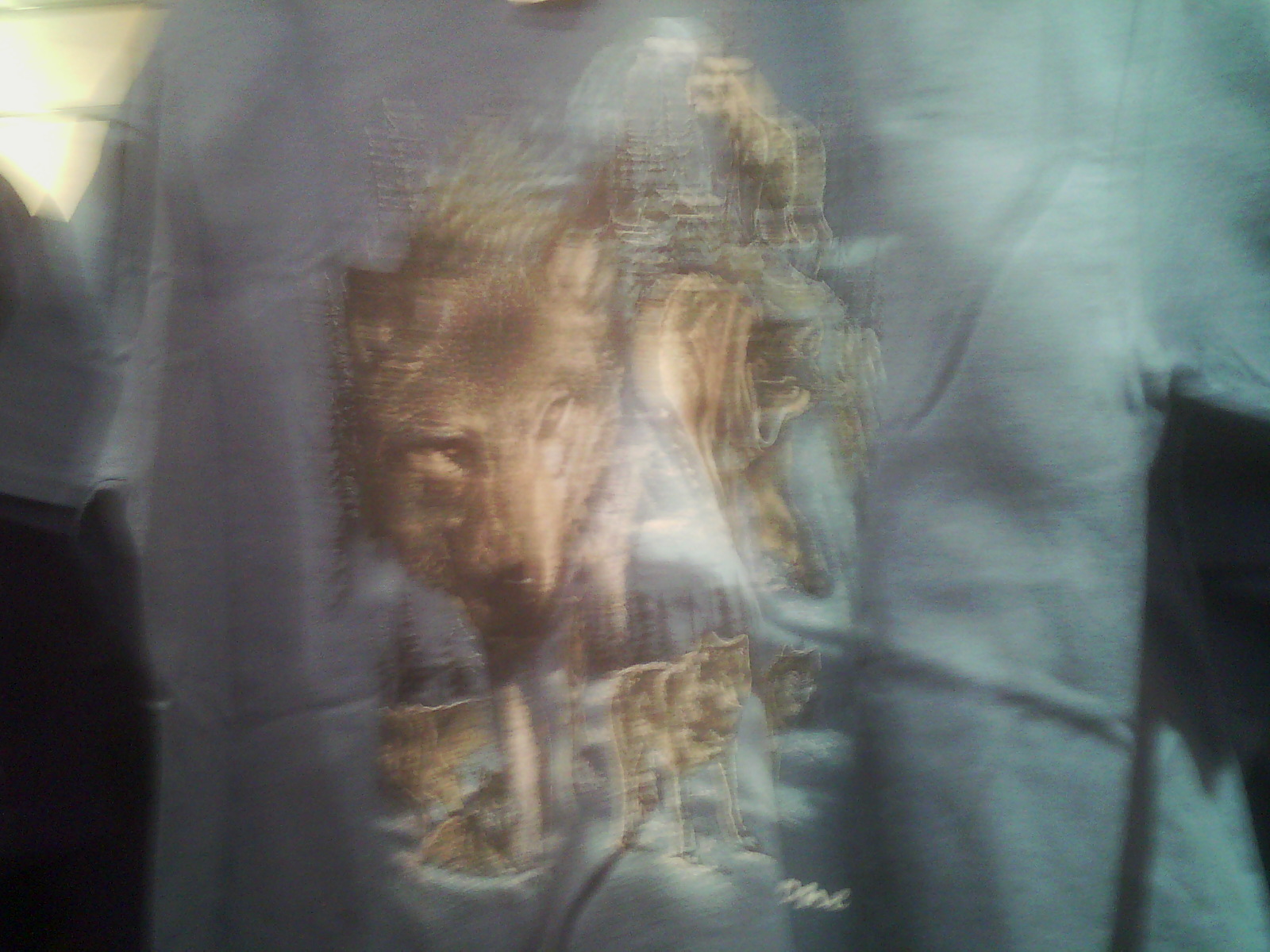This image features a close-up view of a gray, short-sleeve t-shirt, which appears to be laid flat, possibly on a rack or display and not worn by someone. The photo is slightly blurry, adding a bit of ambiguity to the scene. The t-shirt showcases an intricate design of wolves, with one wolf prominently placed front and center, staring directly ahead. Behind it, another wolf is depicted howling at the moon, lending a dramatic, stylized touch to the artwork. In the foreground, a pack of wolves can be seen amid a backdrop of trees, their exact species indeterminate but likely gray wolves or possibly coyotes. The shirt has notable wrinkles, suggesting it was previously folded and has now been unfolded. On the right side of the image, part of the shirt falls into shadow, indicating the presence of another object in the background casting this shadow on the fabric.